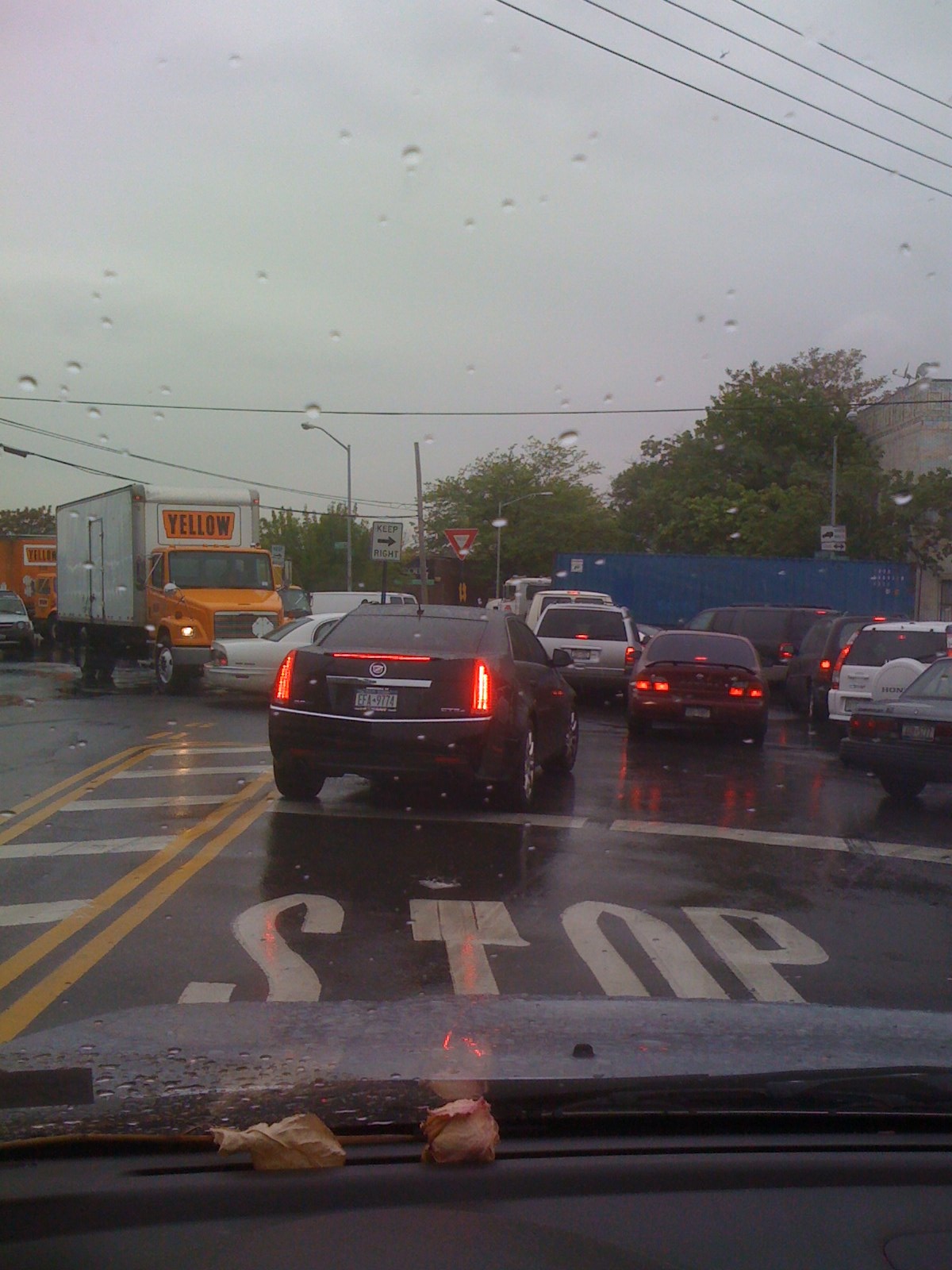This photograph, taken from the driver's perspective inside a car, captures a congested traffic scene at a stoplight. The image looks out through the windshield and showcases a chaotic intersection. At the center, a car attempting to cross traffic is positioned at an awkward angle, with its rear facing the left side of the frame, partially obscured by a nearby black car in the foreground. In the background, a prominent yellow box truck with the word "YELLOW" emblazoned on its side adds depth to the scene. Directly ahead, on the asphalt, the word "STOP" is clearly painted, followed by a thick white line, indicating the stopping point for drivers. The high level of detail in the image emphasizes the complexity and frustration often experienced during rush-hour traffic.